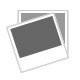This image features a close-up of a glass bottle of powdered creamer laying on its side, showcasing the nutritional facts on the label. The bottle, which resembles an old-fashioned baby bottle, has a creamy yellow plastic cap and is filled to the top with powdered contents. On either side of the bottle, there are two upside-down metal roses, with the left one gold-plated and the right one silver-plated. The background surface appears to be speckled, resembling concrete. The nutritional label on the bottle is partially readable, with details such as 15 calories per serving, 1 gram of fat, 5 grams of sodium, 2 grams of total carbohydrates, and 5 grams of protein. The label also lists directions, stating to add the creamer to hot beverages and limit to four servings daily, and mentions ingredients like coconut oil, milk, and soy. The bottle rests on what seems to be a fabric surface, adding texture to the overall scene.